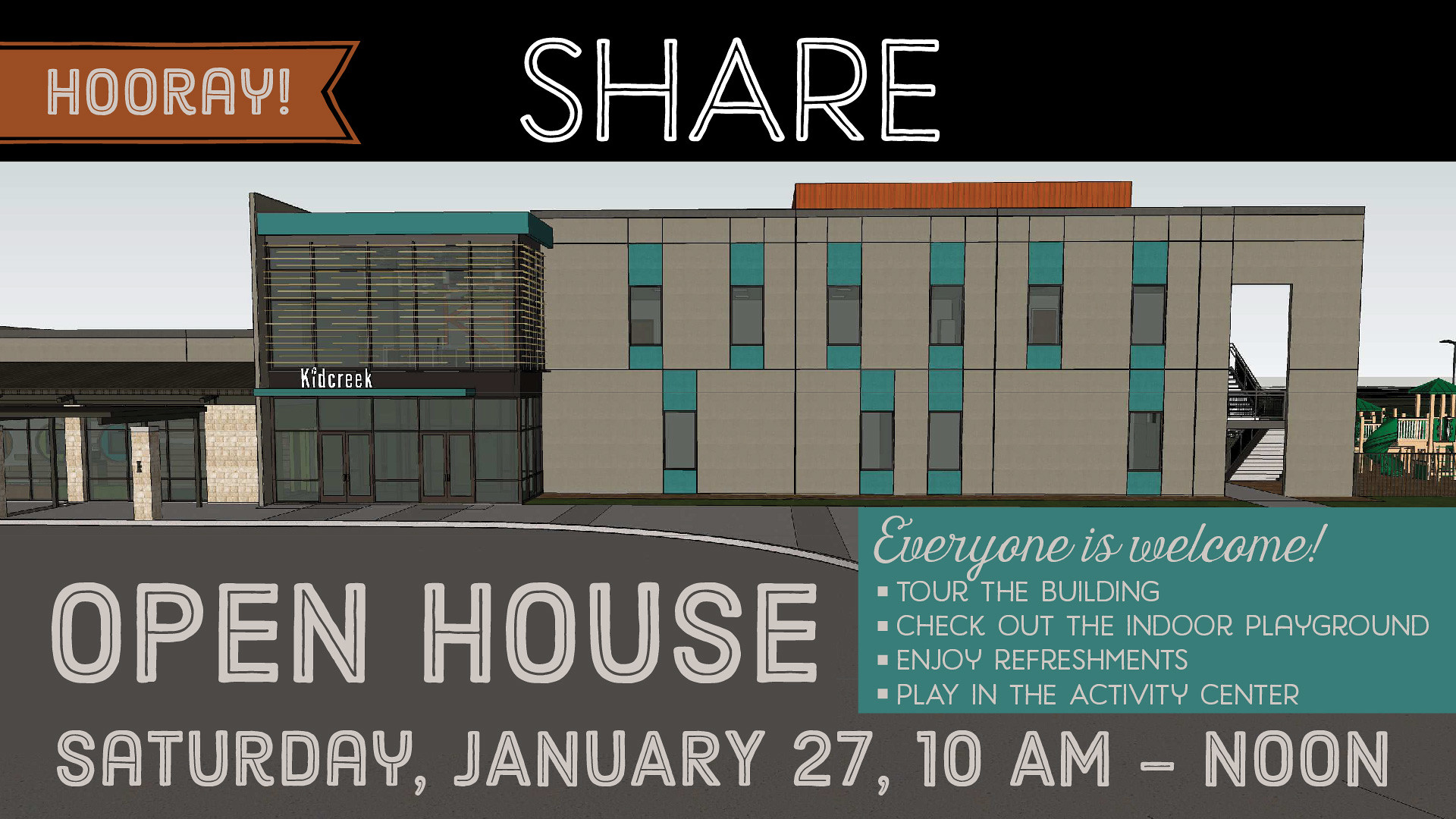This detailed advertisement showcases a horizontally aligned rectangular image. At the top, "HOORAY" is prominently displayed in white letters against a brown background on the left side. Centered beneath a black rectangular background, the word "SHARE" appears in all caps and white letters. Below these headers lies a rendered image of an industrial-looking, multi-story building with gray stonework and blue-accented windows, labeled as "Kid Creek." The building appears slightly unnatural, possibly due to digital rendering.

The bottom portion of the advertisement features detailed event information. A darker gray background displays "OPEN HOUSE" in large white letters, followed by "Saturday, January 27th, 10 a.m. to noon." Between the building's render and the event details, a light blue section with cursive white text announces, "everyone is welcome." Additionally, four bullet points highlight the event's activities: "Tour the building," "Check out the indoor playground," "Enjoy refreshments," and "Play in the activity center."